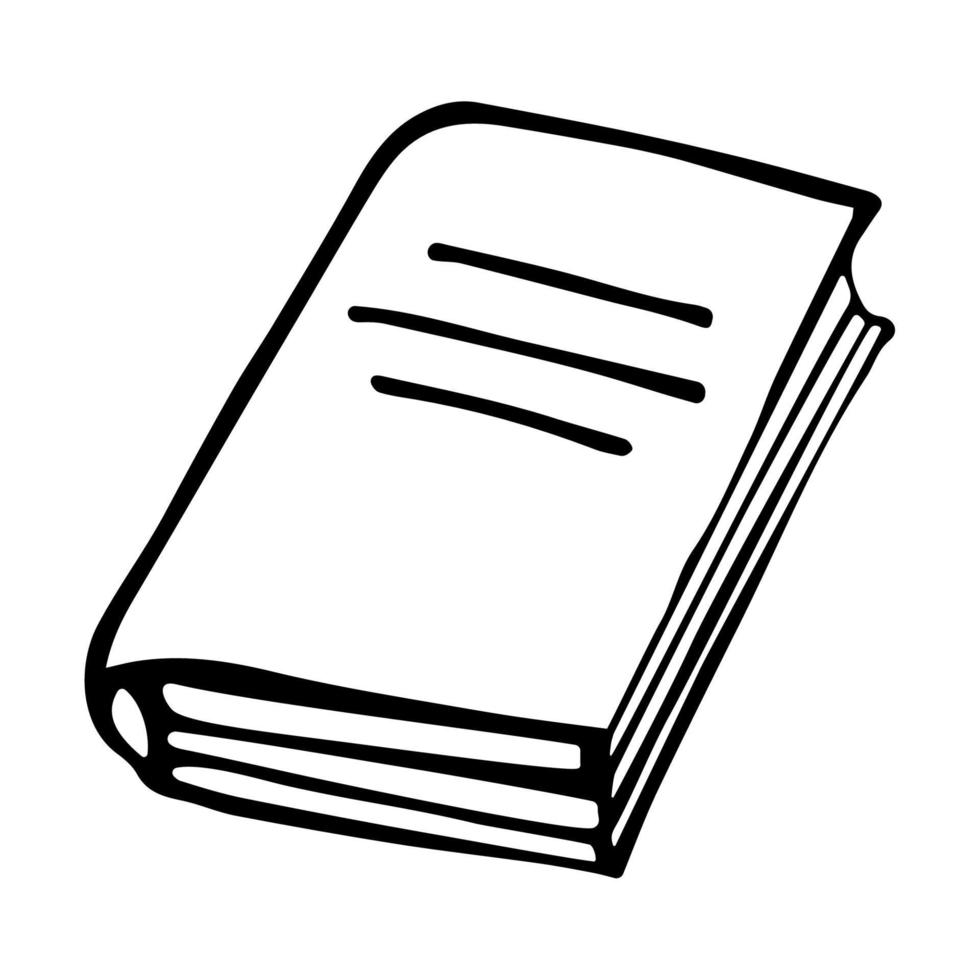The image depicts a simplified, black and white outline drawing of a book set against a bright white background. The book is closed and centrally positioned in the image. It is angled with its top edge facing slightly to the top right and its spine, not visible, oriented towards us and to the top left. The book is primarily white with black outlining, including three thick, black rectangular bars representing the pages on the shorter and longer edges. The front cover features three horizontal black lines of varying lengths, suggesting text or a title. The top and bottom lines are shorter, flanking a longer middle line. There are no objects, text, or numbers in the image, which is crisp and clear, emphasizing the minimalist, monochromatic design.